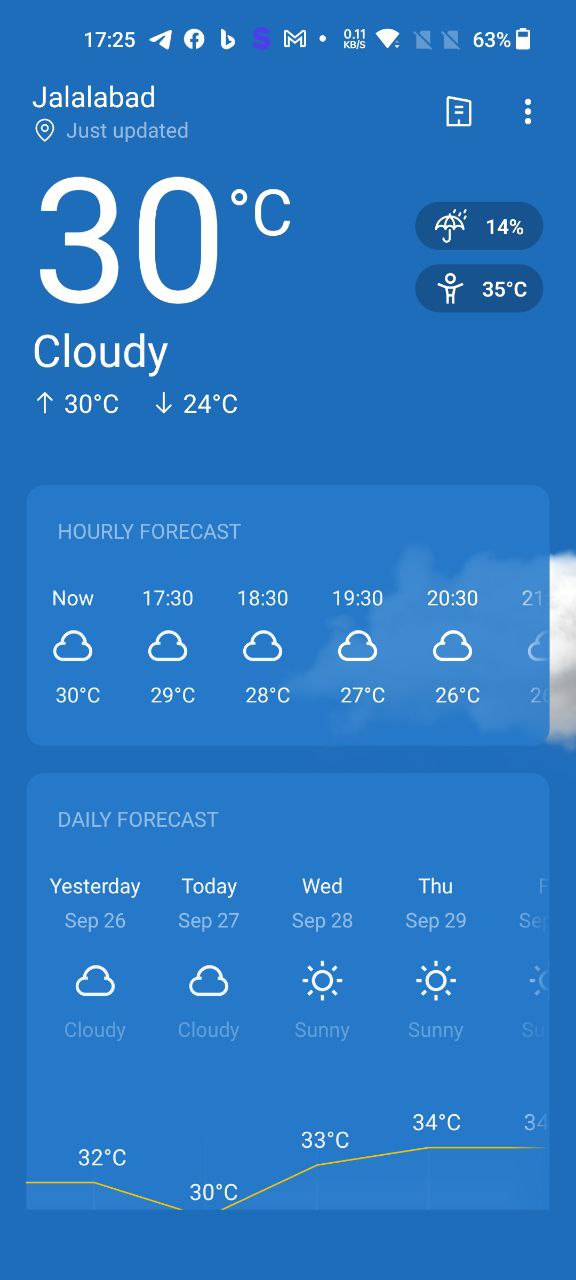This image showcases a detailed screenshot of a weather forecast with a vibrant sky blue background. The screen time displayed at the top is 17:25, accompanied by notifications from Facebook and Gmail, with the device being connected to Wi-Fi and having a battery level of 63%.

The city listed in the forecast is Holabon, presumably located in Asia, followed by a status indicating the forecast has been just updated. The central highlight is the temperature, prominently displayed in elegant gold lettering, marked at 30 degrees Celsius with a current weather condition of 'cloudy'. The detailed forecast also includes a high of 30 degrees Celsius and a low of 24 degrees Celsius.

Below this, the hourly forecast outlines temperature trends for several hours: 17:30, 18:30, 19:30, and 20:30, each showing a gradual decrease from 30 degrees Celsius. The daily forecast is neatly organized in a separate box, covering the days yesterday, today, Wednesday, and Thursday during September. The predictions for the first two days indicate cloudy weather, while the last two days are forecasted to be sunny. A temperature trend line graph at the bottom shows fluctuation from 32 degrees down to 30, then rising again to 33 and 34 degrees.

In the top right corner of the image, a hamburger menu is present along with two icons: an umbrella icon showing a 14% chance of precipitation and a stick figure icon that details a feels-like temperature of 35 degrees Celsius.